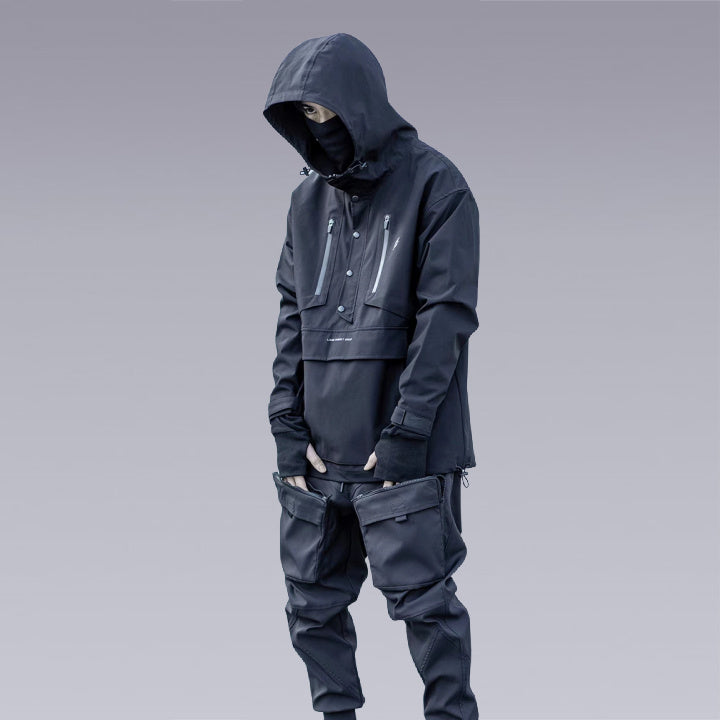The photograph captures a mannequin dressed in a coordinated outfit, consisting of a large, blue hoodie and matching blue pants. The hoodie, which resembles a rain jacket, extends beyond the sides of the mannequin's face, partially concealing it. A black face mask obscures the lower half of the mannequin's face, leaving only the right eye visible, which appears on the left side to the viewer. The mannequin is equipped with fingerless gloves that expose its thumbs and fingers.

The blue hoodie features two vertical gray zippers on either side of the chest, a series of four buttons along the middle, and a closed flap near the stomach area. The pants include two large satchel-like pockets in the front, although the bottom portion of the outfit and the mannequin's feet are not visible. The background transitions from dark gray at the top to light gray at the bottom, creating a stark contrast with the vibrant blue of the clothing.